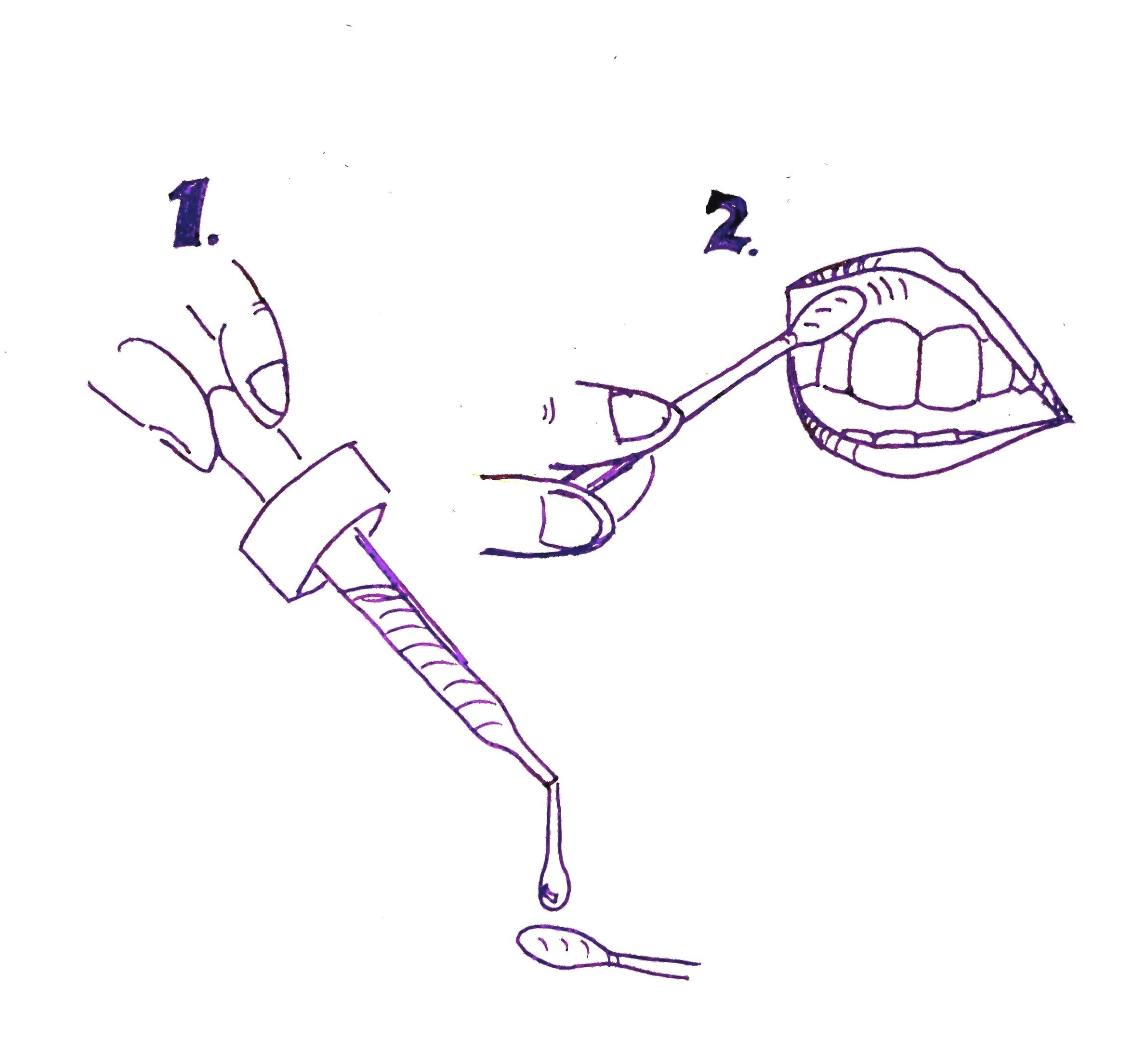The image is a crudely drawn, two-part instructional guide for gum care, primarily illustrated in blue ink with some purple highlights. The first drawing, labeled "Figure 1" with a thickly drawn number "1," shows two fingers squeezing an eyedropper to dispense a drop of liquid onto the tip of a Q-tip. In the second drawing, labeled "Figure 2" with a similarly thick number "2," the same fingers are seen applying the Q-tip to the gumline of an open mouth, just above the front teeth. The simple and unrefined illustrations clearly demonstrate the process of using the dropper to apply liquid to the Q-tip and then rubbing it onto the gums for care or treatment. The repetitive emphasis on the fingers, the eyedropper, and the application to the gumline underscores the instructional nature of the guide.